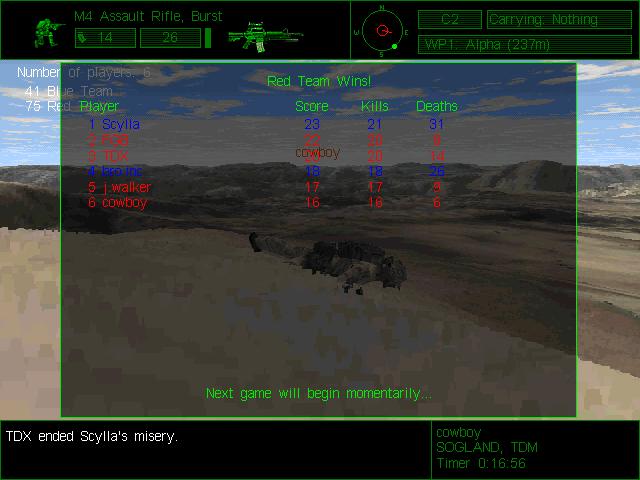The screenshot captures a moment from a video game, highlighting the end of a match. Dominating the center of the image is the game's leaderboard with the vibrant declaration, "Red Team Wins," showcased in green text. The leaderboard lists players' names on the left, accompanied by their scores, kills, and deaths. Just below this, a prompt reassures players that the "Next Game will begin momentarily." 

In the top left corner of the image, partially obscured by the leaderboard, a soldier character is seen lying on a distinctly yellow, pixelated 3D terrain. Beyond the soldier, undulating valleys and hills paint a scenic backdrop. Overlaying this scene is the game's heads-up display (HUD), which details the player's current weapon as an "M4 Assault Rifle Burst," and provides a crouched soldier icon along with the numbers "14 and 26," likely representing ammunition or a score, and an image of the assault rifle itself.

On the top right, a compass HUD element reads "C2, Carrying Nothing, WP1 Alpha," providing navigational and status information. The bottom right corner of the image delivers a succinct combat update with the text "TDX Ended Silla's Misery," indicating a recent in-game event.